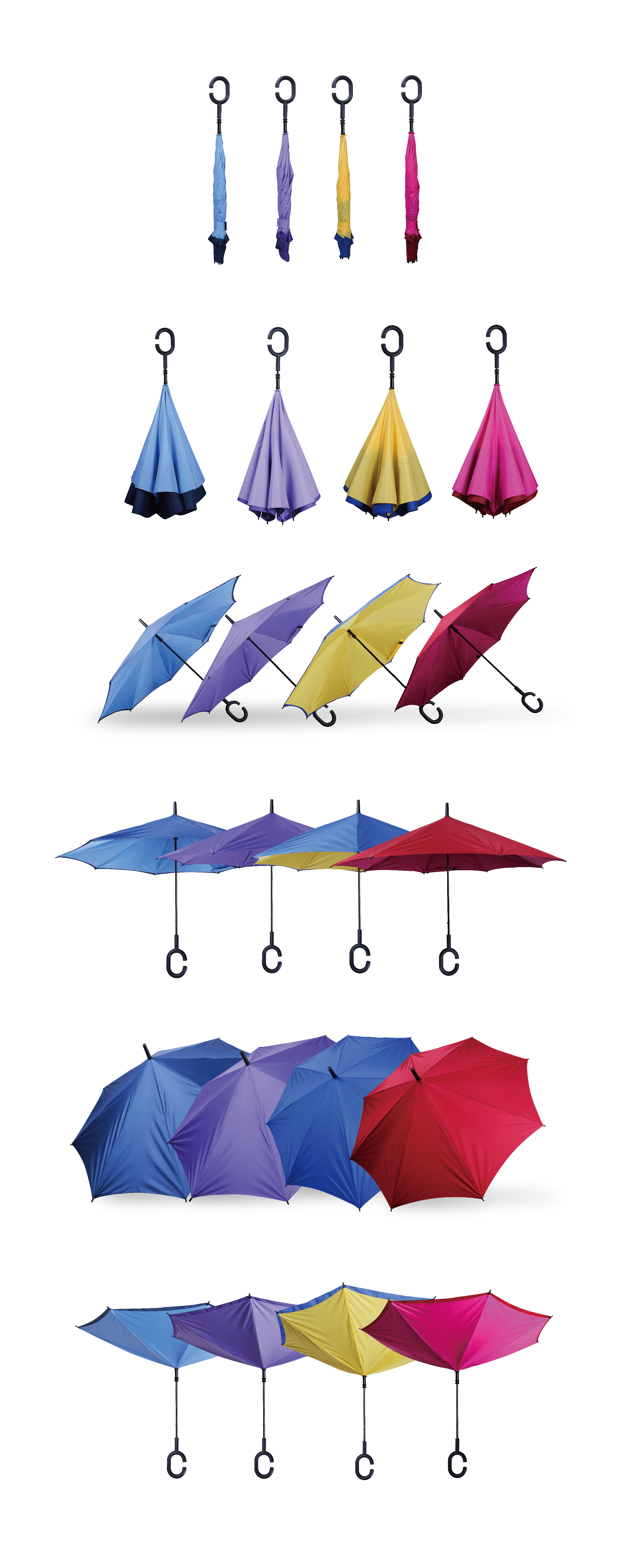This image showcases an advertisement for umbrellas, depicting them in various states of use across multiple smaller images. Each row presents a set of four umbrellas in blue, purple, yellow, and pinkish-red colors. At the very top, a row displays the closed umbrellas, all equipped with a black hook handle. The next row features the umbrellas partially open, beginning to unfurl. Below that, another row shows the umbrellas fully opened and lying at a 45-degree angle with the handles directed to the right. The subsequent row showcases the umbrellas completely open and standing upright, though the support is not visible. Next, the image shifts to a top-down perspective displaying the canopies of the blue, purple, yellow, and red umbrellas. Finally, the last row presents an inverted view of the fully opened umbrellas, highlighting the inside structure with the handles at the bottom. This arrangement effectively demonstrates the versatility and different views of the umbrella products.